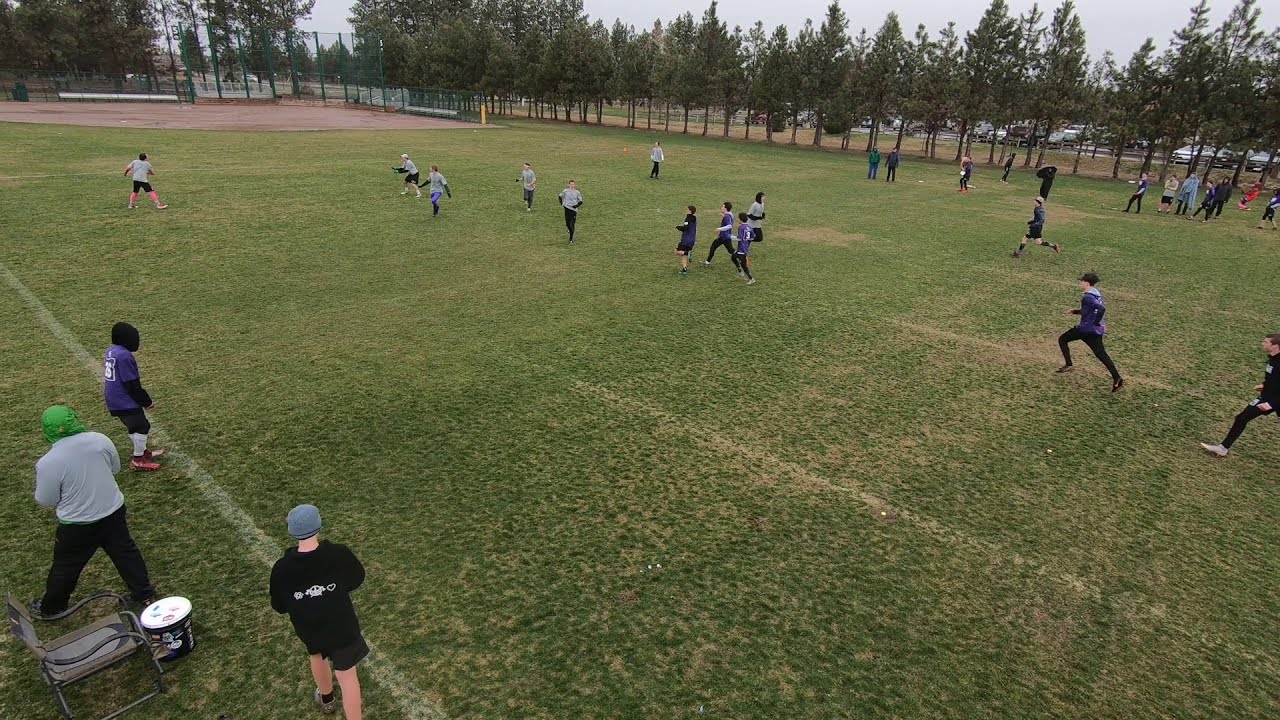In this horizontal rectangular image, we see an amateur soccer game taking place in a large urban park. The setting features a wide grassy field with a goal post visible in the top left corner. Players are divided into two teams, one in white shirts and the other in dark shirts. In the center of the image, children are actively engaged in the game, running, jumping, and playing on the well-manicured turf. Surrounding the park are towering evergreen trees, which line the background and provide a lush, green backdrop. A baseball diamond, with its characteristic dirt, is faintly visible at the far end of the park.

Along the sideline to the left, a coach, distinguishable by his green cap, light shirt, and dark pants, stands with a couple of players who are waiting to join the game. Nearby, there is a chair and a stool. To the right, some spectators, possibly parents, are gathered to watch the game. Beyond the trees to the right is a parking lot filled with cars, presumably belonging to the players' families. The scene is set under an overcast sky, casting a diffused light over the vibrant green, brown, gray, and occasional bursts of red, purple, and yellow colors scattered throughout the image.